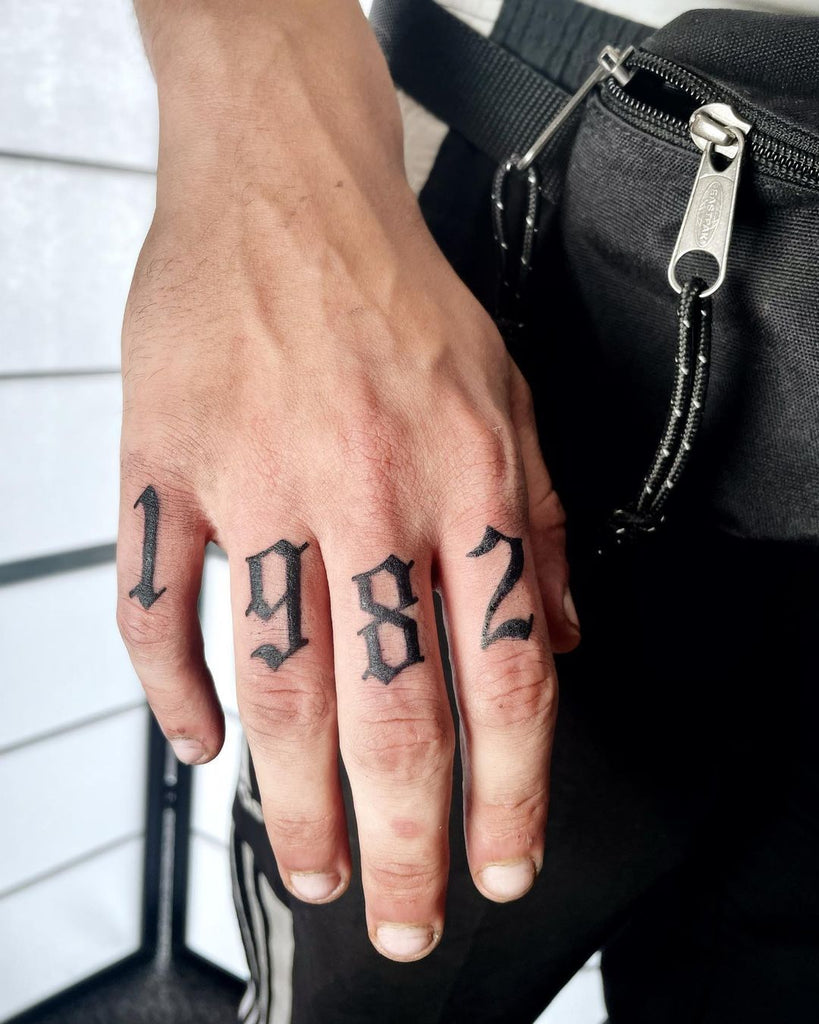This color photograph captures a close-up of a person's right hand extending from the top of the frame. The hand, slightly veined with a hint of hair, displays short nails and features tattoos across the knuckles spelling out the year "1982" in black, gothic-style text, starting with '1' on the pinky and ending with '2' on the index finger. The person is dressed in black pants, which bear three white stripes down the side, hinting at a possible Adidas brand. A black fanny pack with two silver zippers, one partially unzipped and adorned with a small braided fabric pull, sits around their waist. The edge of a white shirt peeks out slightly above the waistline on the top right. The background is a bright, white wall, possibly consisting of hinged, movable privacy screens. The photograph contains no additional writing, animals, mechanical objects, or motorized vehicles.